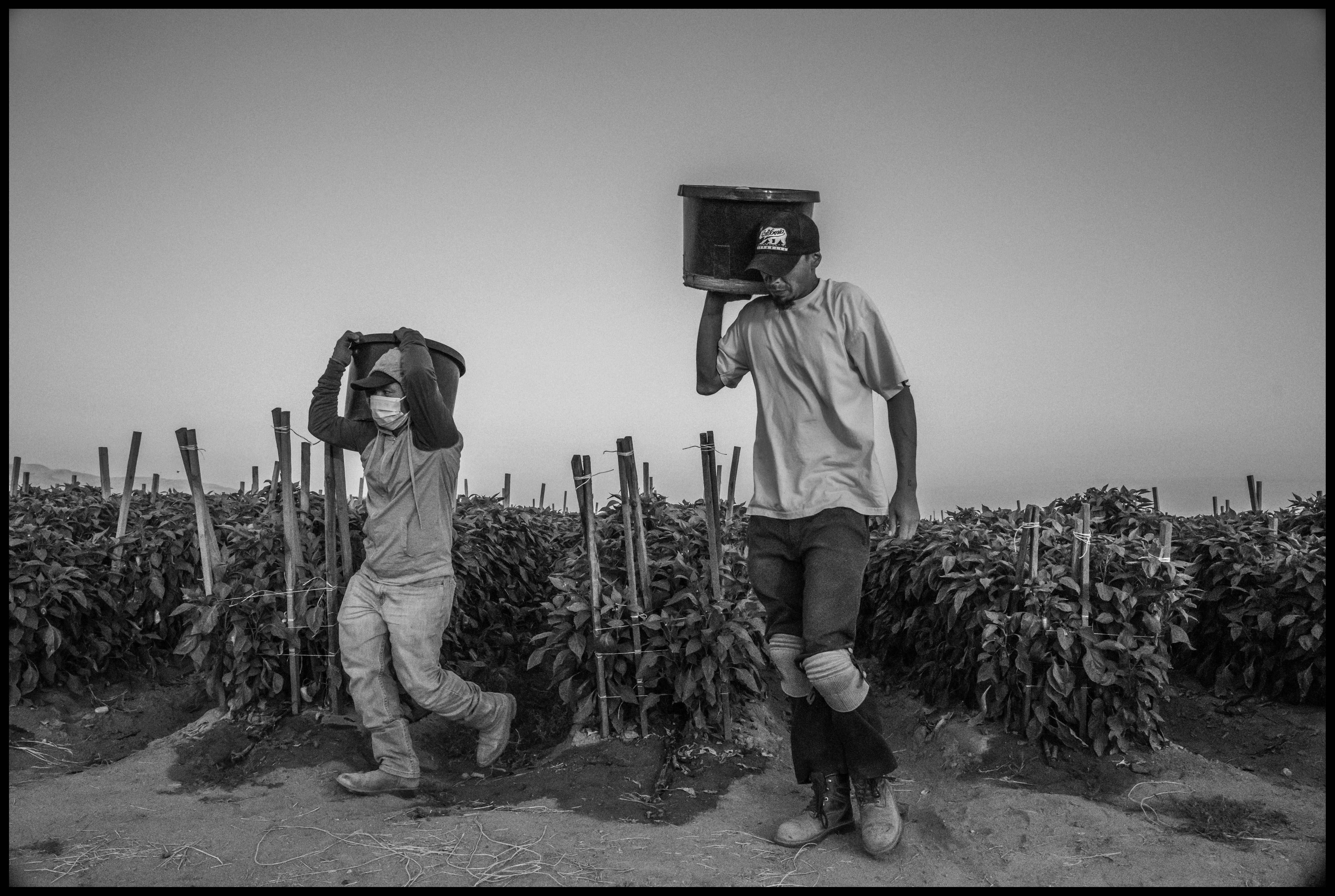In this horizontally aligned, black-and-white photograph framed by a thin black border, two men, dressed in work attire, are depicted as harvesters emerging from rows of crops that stretch across the foreground. The entire scene rests on a dirt ground with plants supported by wooden sticks protruding upwards. The backdrop is a sky blending light and medium gray tones.

The man on the left, shorter and stockier, wears a dark long-sleeved shirt with a hood, a black baseball cap, a white face mask, and rugged high-top boots. He's also sporting dirty pants and carries a large black bucket on his right shoulder. The taller man to his right, contrastingly slender, dons a dirty white T-shirt, jeans, knee pads, and hiking boots. He grips a black bucket with one hand, raising it above his head with some assistance from other boys. 

Both men are traversing one of the four visible rows of crops. At least six rows can be seen extending far into the background, under a gray sky, making a visually harmonious scene of diligent labor amid the crop fields.